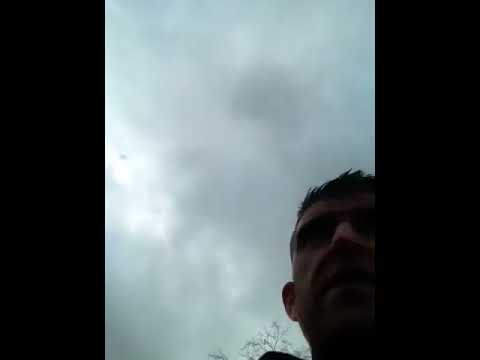The image depicts a dimly lit, outdoor scene predominantly featuring a gloomy, overcast sky filled with gray and darker gray clouds, suggesting impending rain. Positioned in the lower right-hand corner is a white man, viewed from below from approximately chin height, making his face appear offset. His facial features are largely obscured due to the dim lighting, rendering his eyes and mouth almost indistinguishable. He has short black hair, shorter on the sides and slightly longer on top. Visible on the left side of the image, just behind the man, is the top of a leafless tree, its branches stark against the cloudy sky. A small black area, possibly his shoulder or part of a garment, is also visible. The image has thick black borders on both the left and right sides. The overall atmosphere of the photo is dark, gloomy, and minimalist.